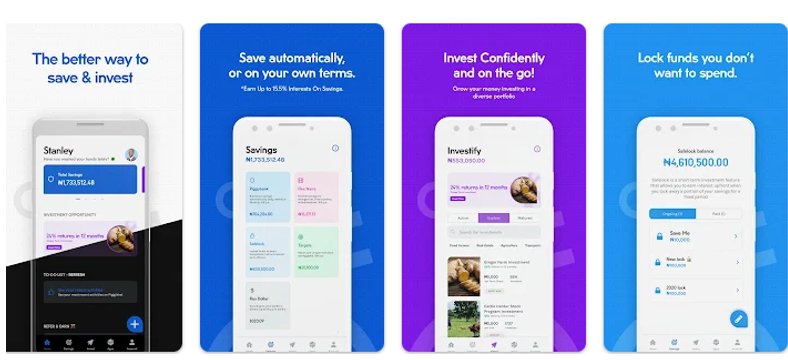The provided image is a screenshot of an application showcasing various features through four distinct, brightly colored sections.

1. The first section has a white background with blue text that reads, "The better way to save and invest." It features an image of a smartphone displaying the app interface, with the word "Stanley" prominently visible. The interface also includes a blue bar, alongside purple and gray writing set against a black background.

2. The second section emphasizes automatic savings options with the phrase "Save automatically or on your own terms" set against a blue background. It highlights an opportunity to earn up to 15% on savings. A depiction of a white smartphone shows the app's savings feature, with various colored squares (blue, red, green, light blue, and gray) representing different components of the savings.

3. The third section encourages users to "Invest confidently and on the go" against a purple background. The smartphone screen displays the text "Invest, Investify," with purple writing and images depicting the various investment options available within the app.

4. The fourth section advises users to "Lock funds you don’t want to spend," reinforcing the functionality of managing finances effectively.